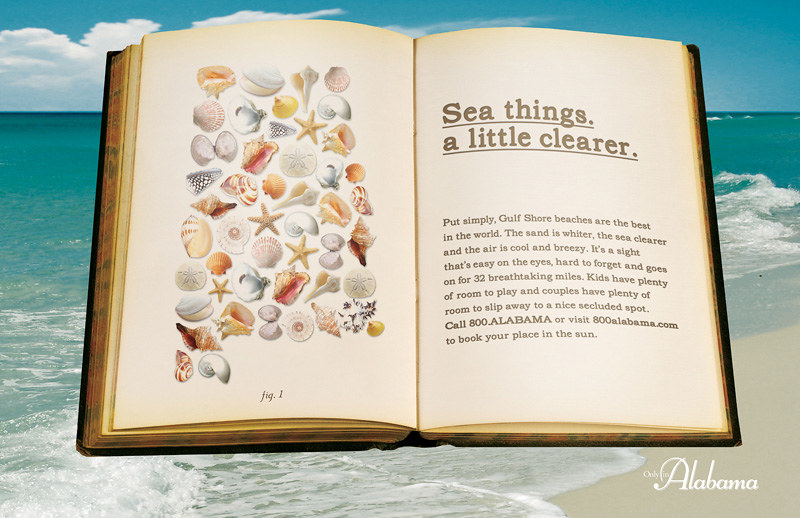The photograph features a picturesque beach landscape as its backdrop, with the perspective from the sandy shore looking out towards the vibrant horizon. The beach sand is of a very light, nearly white hue, adorned with gentle waves that lap at the shore. The ocean transitions from a serene light green near the foreground to a darker blue as it approaches the horizon, under a sky dotted with a few clouds.

Centrally imposed on this serene scene is the image of an open brown book. The book is open towards the back third, with its left page displaying an assortment of seashells arranged in a neat rectangle, featuring a variety of shapes and colors, including clam shells and starfish. The right page contains descriptive text in brown letters that begins with the phrase, "See things a little clearer," with "Sea" cleverly spelled as "S-E-A." This is followed by an advertisement: "Put simply, Gulf Shore beaches are the best in the world. The sand is whiter, the sea is clearer, and the air is cool and breezy. It's a sight that's easy on the eyes, hard to forget, and goes on for 32 breathtaking miles. Kids have plenty of room to play, and couples have plenty of room to slip away. It's a nice secluded spot."

Additional contact information is also provided at the bottom of the right page, encouraging viewers to call 800-ALABAMA and visit 800alabama.com to book a visit. The overall composition of the image suggests a promotional ad for the Alabama Gulf Shore beaches, combining the tranquil beach setting with the inviting text from the book to convey a compelling message.